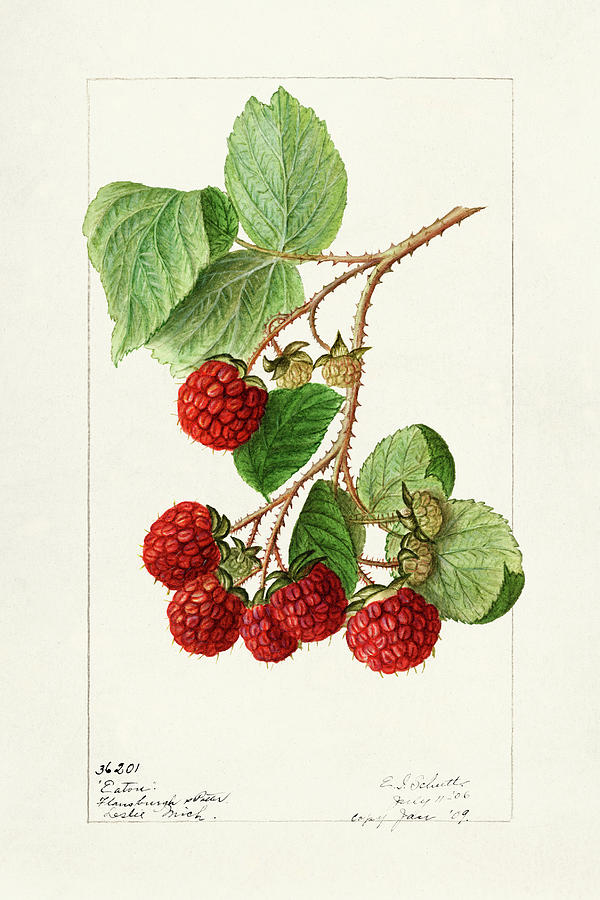This detailed botanical illustration of raspberries is set against a beige, off-white background, framed by a thin dark gray border. The painting prominently features a thorny vine that enters from the right side, branching out in various directions. Atop the branches are six bright red ripe raspberries, complete with tiny seed details and hair-like structures typical of raspberries. In addition, there are several smaller, tan-colored unripe berries. The vine and its offshoots are adorned with a mix of bright to light green leaves, some larger and variegated, each showing detailed vein work.

The vine’s stems are spiked with short, stocky thorns, adding a tactile quality to the image. Below the berries, some leaves bend and fold naturally around the vine. In the bottom left and right corners of the image, handwritten text in cursive is visible, though mostly illegible except for the number "36201." The text also seems to include partially legible words such as "eaten" and possibly "Leslie, MICH". The year "09" is faintly discernible, suggesting an older date. This detailed rendering effectively combines the precision of botanical illustration with the evocative qualities of vintage artwork.